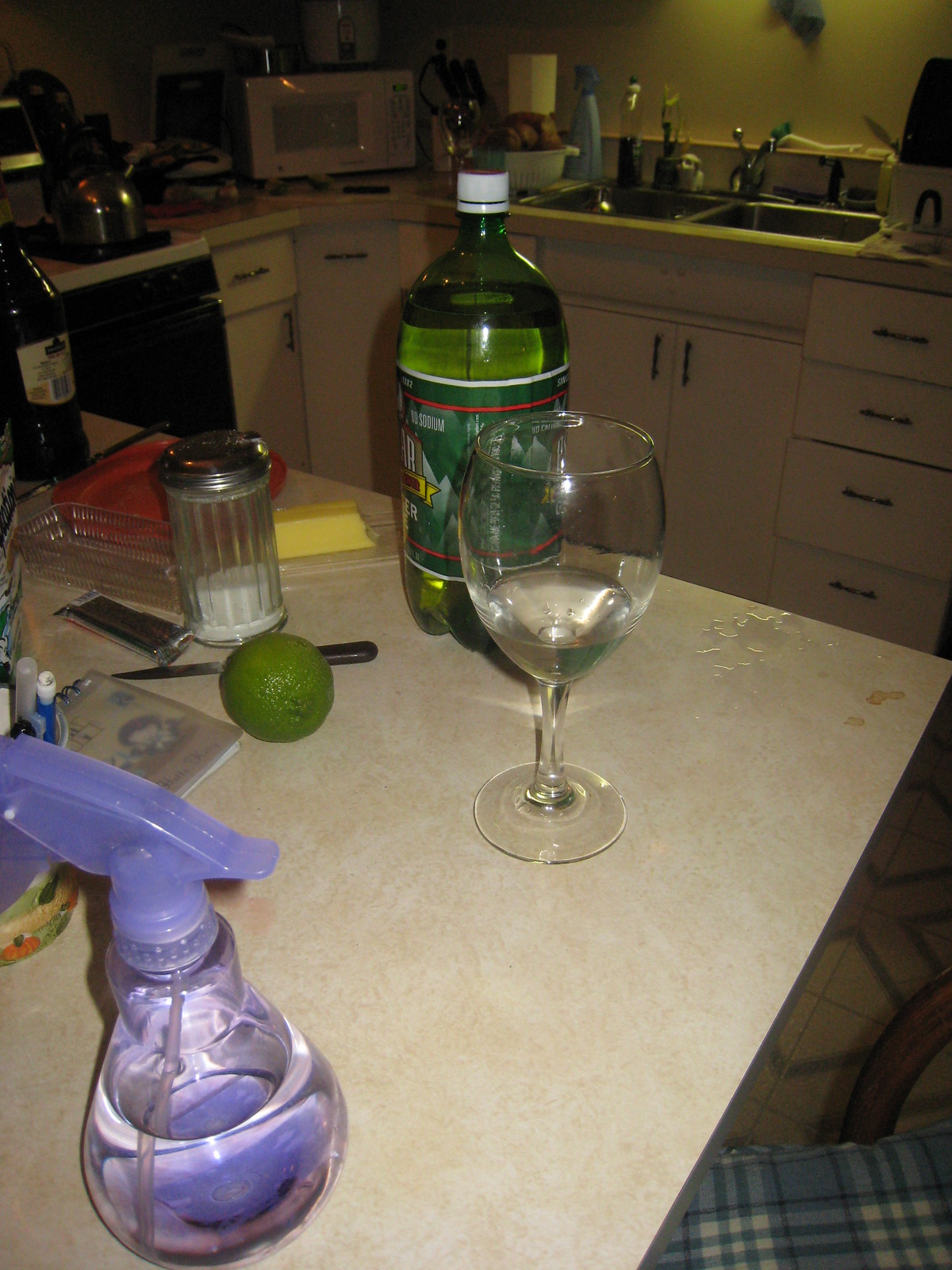This image captures a cluttered table with various items arranged across its surface. Closest to the viewer, on the left, is a spray bottle with a purple top and clear bottom, containing a transparent liquid. Moving upward, there is a small notebook, a lime, and a classic diner-style container likely holding sugar. Alongside these items lies an upside-down granola bar and, further to the left, a jar filled with pens. In the background, a bottle resembling triple sec stands partially obscured. To its right, a red Tupperware lid is positioned beside an open-faced stick of butter. Further right, an unopened two-liter bottle of Polar Brand ginger beer stands next to a quarter-filled wine glass, likely containing white wine. A spill of clear liquid is visible on the table's surface, and the scene is set against a dimly lit kitchen in the background.